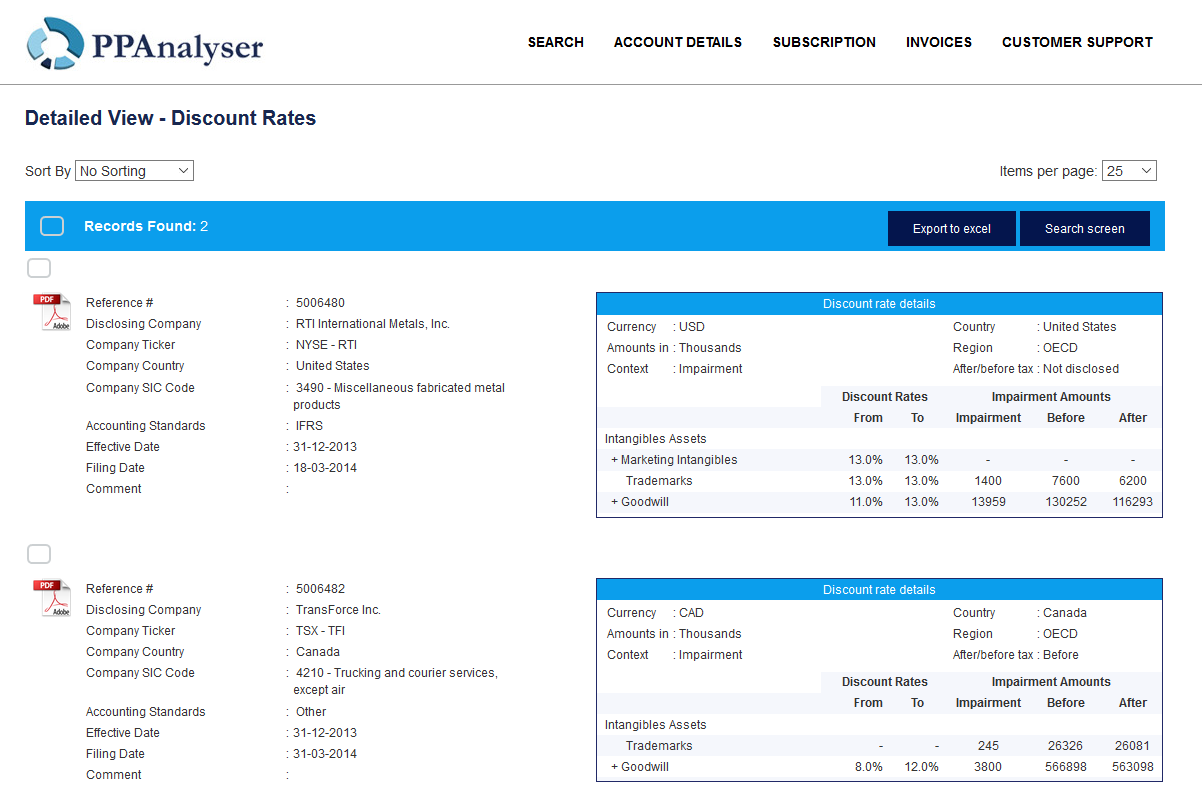The webpage features a detailed interface for the "PP Analyzer." At the top left, there's an aqua blue logo with the text "PP Analyzer" adjacent to it. Centrally aligned at the top of the page are menu options: "Search," "Account Details," "Subscription," "Invoices," and "Customer Support."

Beneath the navigation line, on the left side, there's a section titled "Detailed View - Discount Rates." Here, there's a sort drop-down menu, which is currently unselected. On the far right of this section, there's another drop-down for "Items Per Page" showing 25 items are currently selected.

Below this section is a light blue banner indicating "Records Found: 2." On the far right of the banner, there are two darker blue buttons with white text: "Export to Excel" and "Search Screen."

The main content area displays two records. Each record begins with a PDF icon on the left. To the right of the icon, columns list the reference number, disclosing company, company ticker, company country, SIC code, and various other details. On the far right of each record, there's a square box containing detailed information about currency amounts and accounts. The layout for both records is consistent, with each detail methodically organized to offer comprehensive information at a glance.